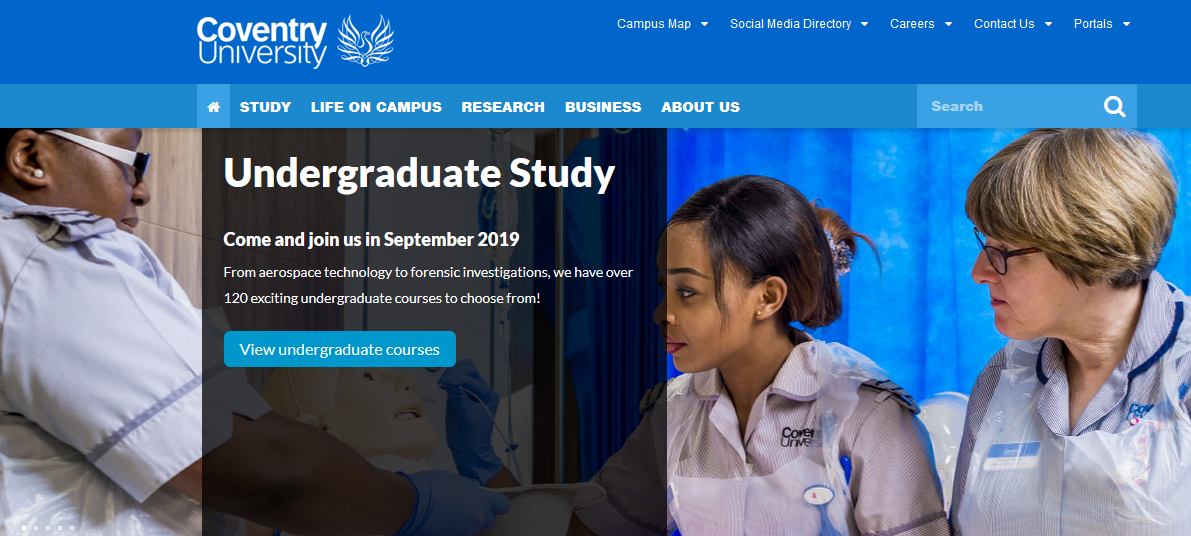The image showcases a webpage from Coventry University's official website. At the top, there's a dark blue banner featuring the text "Coventry University" in bold, white print with the "C" capitalized. Adjacent to the text is a graphic logo resembling a bird with wings extended on both sides.

Moving to the right section of this banner, there are several menu options, each with a drop-down feature: "Campus Map," "Social Media Directory," "Careers," "Contact Us," and "Portals."

Below this, a lighter blue banner spans the width of the page, containing navigation links in white text: "Home," "Study," "Life on Campus," "Research," "Business," and "About Us." A search bar with a white magnifying glass icon is also present for user convenience.

Dominating the main section of the page is a graphic image. It depicts a woman wearing sunglasses and pearl earrings, focused on the right side of her face. She is dressed in what appears to be a short-sleeved shirt or uniform. Next to her is another individual, also in a uniform, working on a mannequin. 

Overlaying this graphic is text promoting undergraduate studies: "Undergraduate Study: Come and join us in September 2019. From aerospace technology to forensic investigations, we offer over 120 exciting undergraduate courses to choose from." 

At the bottom of this section is a call-to-action button, presented on a blue banner with white text that reads, "View Undergraduate Courses."